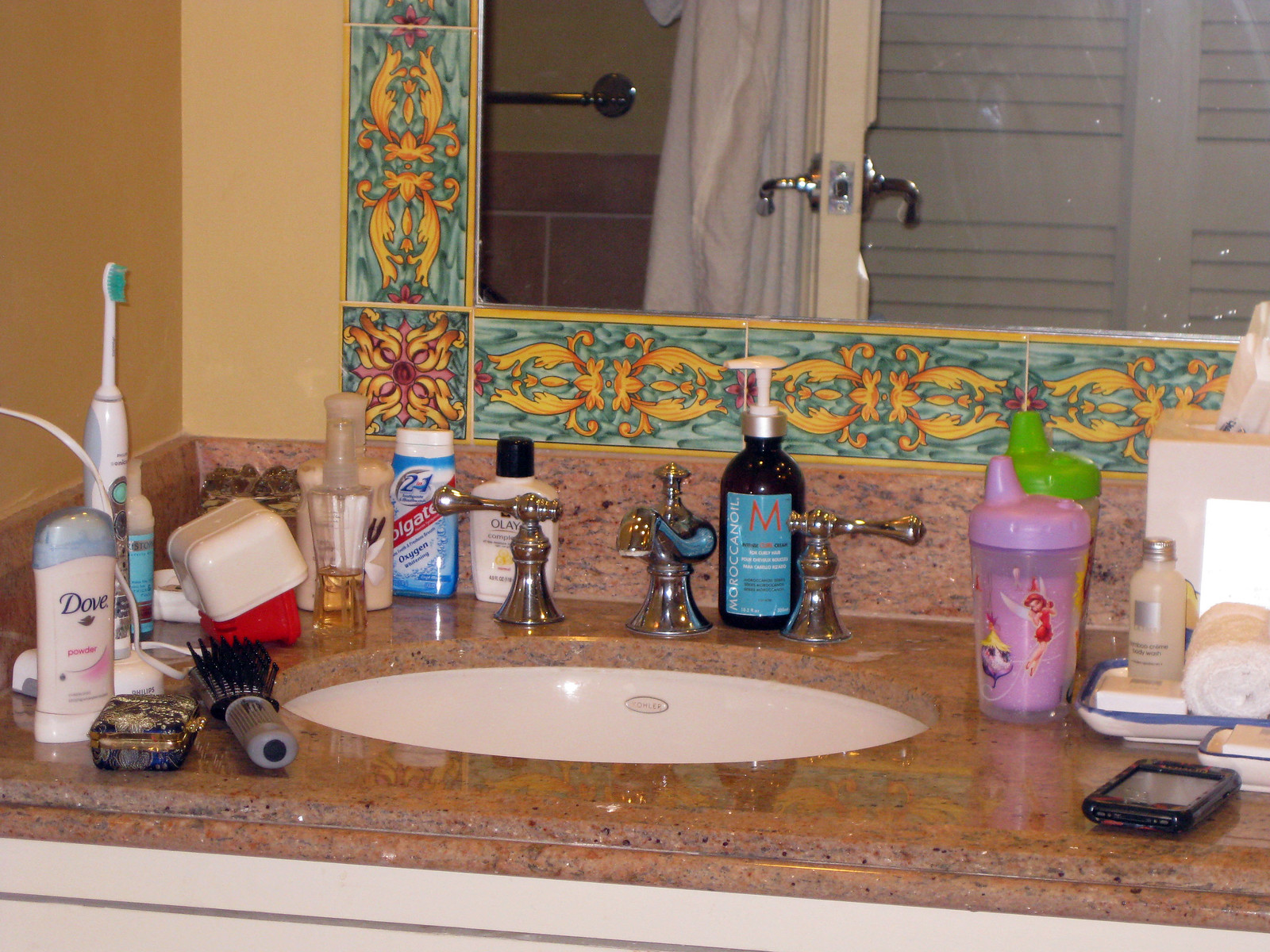The image is a color photograph capturing a detailed view of a bathroom sink counter. At the center of the scene is a round sink accompanied by stainless steel faucet fixtures. The countertop, fashioned from brown granite, gleams with reflections of the surrounding faucet and assorted items, indicative of its polished surface. Positioned against a dark yellow wall to the left, the sink counter showcases an array of healthcare and makeup products scattered around. Among these items, identifiable objects include a Dove deodorant, an electric toothbrush, a container of Q-tips, toothpaste, a bottle of liquid soap, two sippy cups, and a neatly arranged tray of makeup.

The backsplash portion of the wall behind the sink is adorned with intricately patterned tiles that feature a mix of yellow, red, and greenish-blue hues, adding a vibrant touch to the space. Above this, a mirror framed by the same colorful tiles hangs, reflecting additional elements of the bathroom. In the mirror's reflection, one can see the edge of a door complete with its doorknob, a closed cabinet to the right, and a shower equipped with a metal shower bar to the left. The overall image offers a comprehensive glimpse into the bathroom's well-appointed and colorful setting.